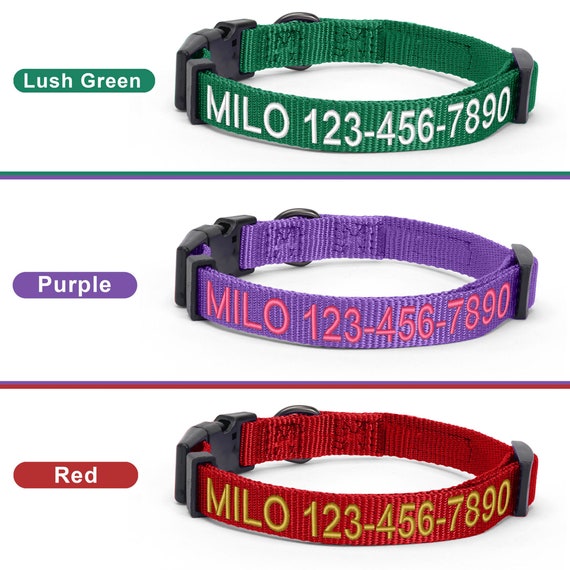The image depicts a set of three customizable dog collars displayed against a white background. Each collar is showcased horizontally, one above the other, forming a vertical trio. At the top, the first collar is labeled "Lush Green" on the left side in matching green text and features white lettering that says "MILO 123-456-7890." The green collar displays a sleek, vibrant appearance.

Beneath it, the second collar is presented in a rich purple hue with the label "Purple" on the left in purple text. It displays the same "MILO 123-456-7890" text but in pink lettering, providing a distinct contrast against the darker material.

The third collar at the bottom is in a deep red color, labeled "Red" on the left in corresponding red text. This collar also features the "MILO 123-456-7890" text, but with letters in a gold or brownish color.

Each collar includes a buckle and an adjustable component, indicating the high-quality fabrication and bespoke nature of the product. The clear segmentation by color and comprehensive detailing underscore the collars' customization options available for purchase on the retail website.